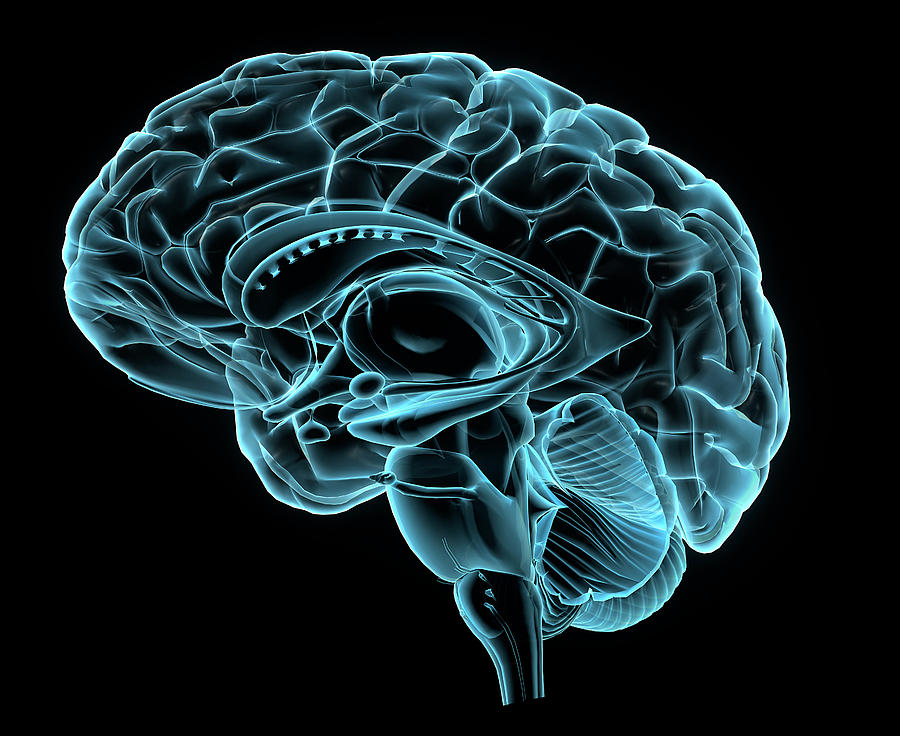The image features an intricately detailed, computer-generated illustration of a human brain on a completely black background. The brain is depicted in a stylized, translucent, electric blue color, allowing visibility of its inner structures and contours. The brain is presented from a side view, with the frontal lobe on the left and the brainstem on the right, extending to the bottom of the image. The digital rendering highlights various anatomical features, such as veins, arteries, and possibly the pituitary gland, all depicted in shades of blue and green. The image also includes swirling patterns and a notable circular area in the center, adding to the visual complexity. The overall effect is a neon, fluorescent glow, providing a rich contrast against the dark backdrop, emphasizing the brain’s morphology and intricate details.